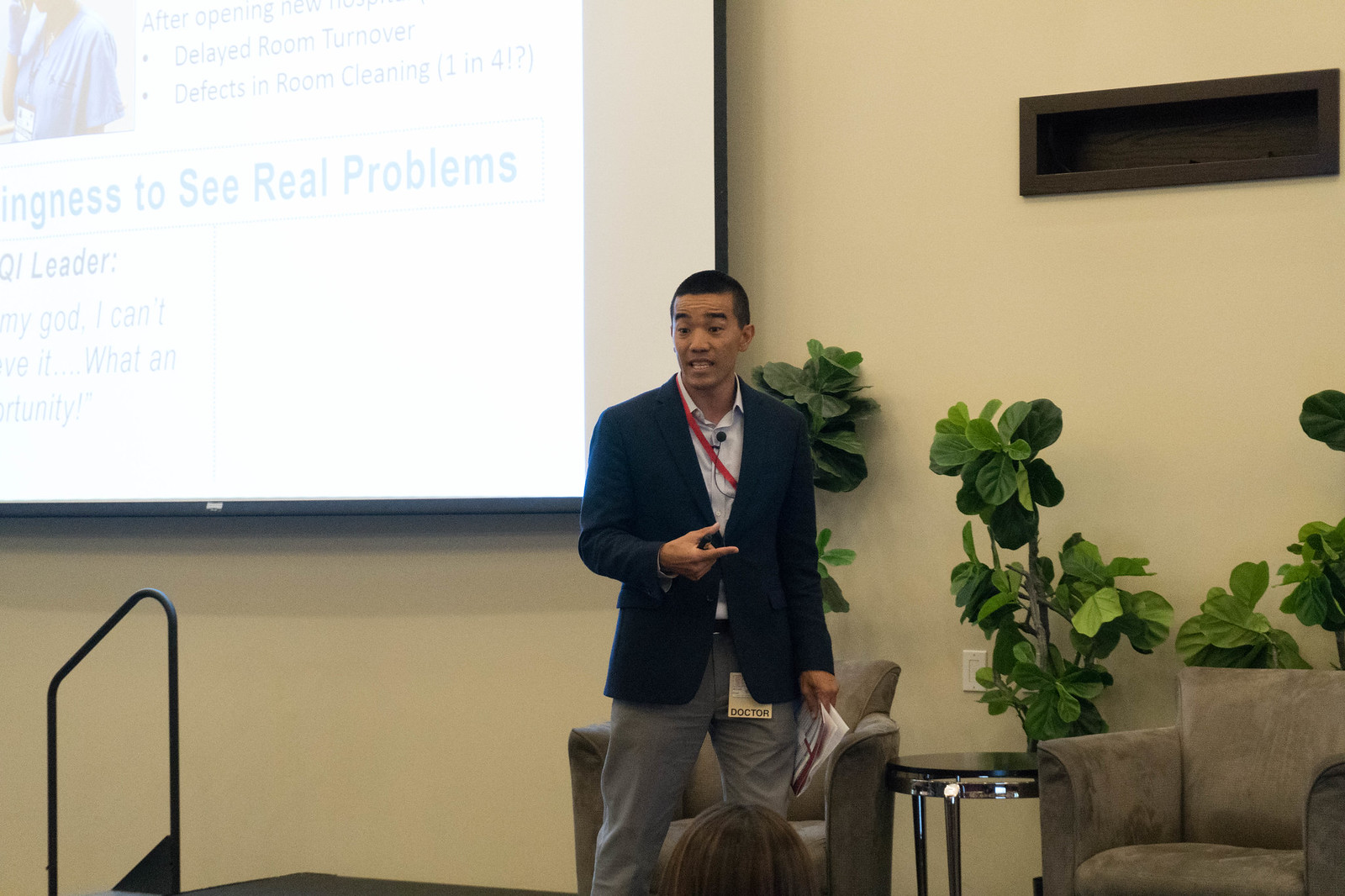The image is a detailed photograph of a man, possibly of Asian or South American descent, giving a presentation at a conference. He is standing mid-sentence on a raised platform equipped with a black ramp and railing on the left side. The man is wearing a light blue button-down shirt, a dark blue jacket, and gray slacks. He is also adorned with a red lanyard and badge that identifies him as a doctor or director, with a lanyard microphone clipped just below his collar. 

Behind him, the setup includes two gray fabric armchairs with a round, glossy black table between them, and potted plants adding a touch of greenery. The wall behind him is off-white and features a partially visible presentation slide with blue text, snippets of which read, "operating new delayed room turnover defects in room cleaning one in four willingness to see real problems leader." Part of a woman's head and hair is visible, indicating an audience in attendance. Additionally, the image captures part of a black dolly in front of the speaker, suggesting equipment used for the presentation.